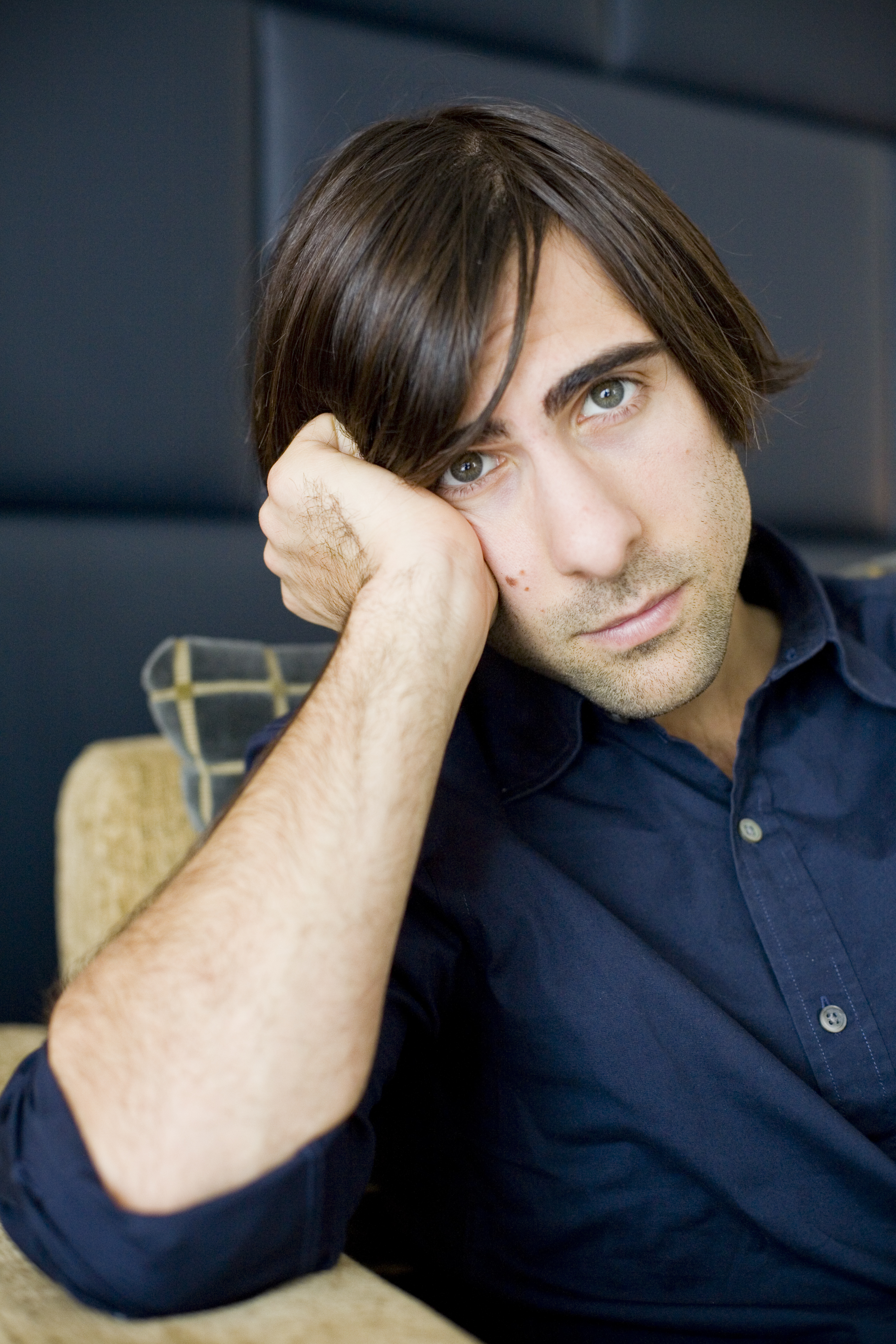This is a vertically aligned rectangular photograph of a man, possibly in his 20s or 30s, who appears to be Jason Schwartzman. He has straight, short brown hair swept to the side and is wearing a navy blue button-up shirt with the sleeves rolled up. He is seated in a tan chair with a gray and gold cushion on the back and a gray pillow with small tan straps behind him. His right elbow rests on a table or counter, and his right wrist is leaning against the right side of his face near his eye, with his fingers folded back. He has slightly gray eyes and a neutral expression, looking directly at the camera with his mouth closed. The wall behind him is made up of large, dark gray blocks, resembling a padded headboard.